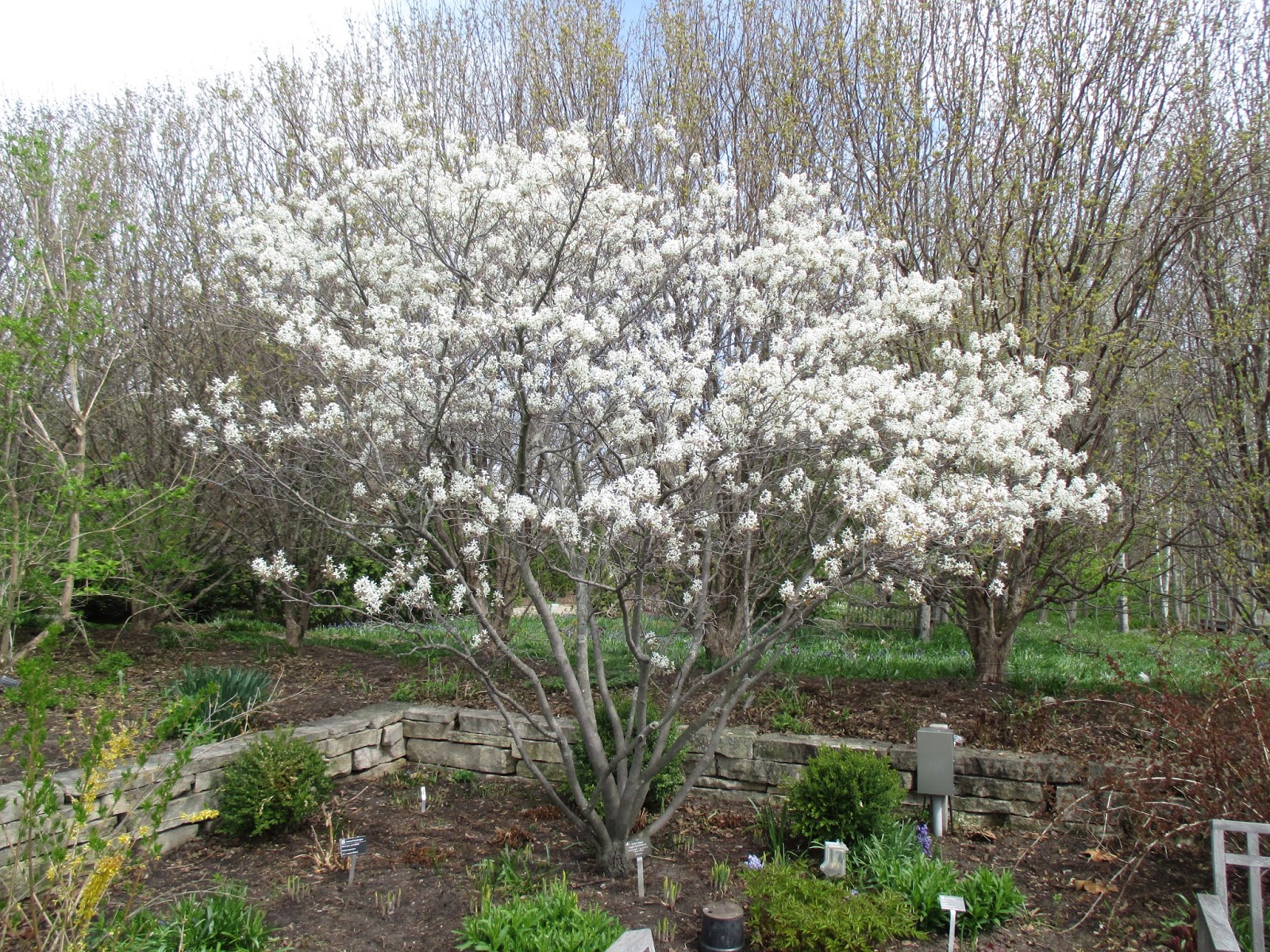The image, likely taken in the daytime at a botanical garden, prominently features a tree with white flowers, centrally positioned in a landscaped area. The tree has a gray trunk that branches out in a V-shape, adorned at the tips with delicate white flowers. Encircling the tree is a miniature brick wall that contains various shrubs and smaller plants, each marked with small, unreadable labels. This section of the garden also includes mulch and some scattered signs and small lights planted in the ground.

Beyond this focal point, the background reveals a vibrant garden scene with expansive green grass and an assortment of trees, some budding with green leaves as if in early spring, while others appear dry. The sky overhead is a patchwork of blue and white, indicating a partly cloudy day. In the distance, benches and more greenery detail this lush, meticulously maintained environment. The scattered positioning of elements throughout the image accentuates the natural yet thoughtfully designed layout of the garden.